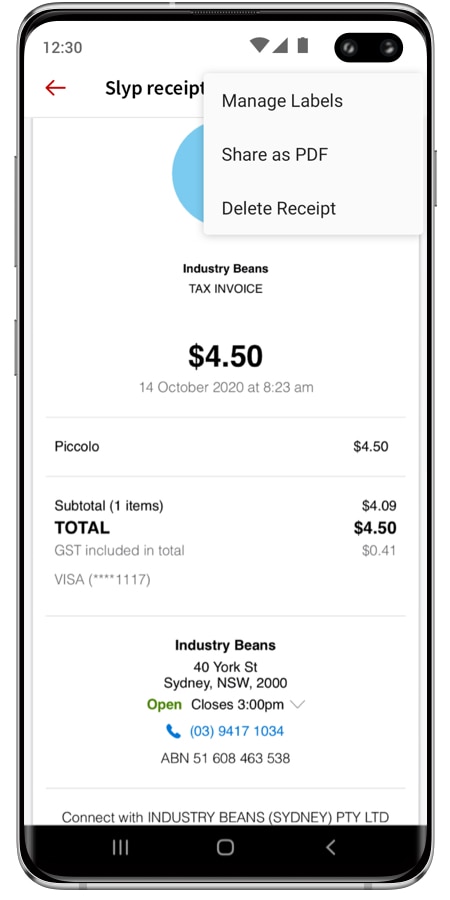**Caption:**

The image captures an active screenshot on a smartphone displaying a digital receipt from Industry Beans. The phone, with its black bezel, is shown suspended against a white background, settled in an upright position. At the top of the screen, a gray drop-down menu provides three options: "Manage Labels," "Share PDF," and "Delete Receipt." This menu partially obscures the top of the receipt.

The receipt is titled "S-L-Y-P Receipt." Below the drop-down menu, the receipt features a prominent blue circle followed by the text "Industry Beans Tax Invoice." Central to the display, the amount $4.50 is shown, covered by the label "piccolo," indicating the purchase. The receipt's date and time are noted beneath this in small gray font: 14 October 2020 at 8:23 PM.

Further down, the receipt breaks down the purchase details, showing a subtotal and total of $4.50. At the bottom, the contact information for Industry Beans is provided: located at 40 York Street, Sydney, NSW 2000, the café is open until 3 PM, and it lists a phone number for contact.